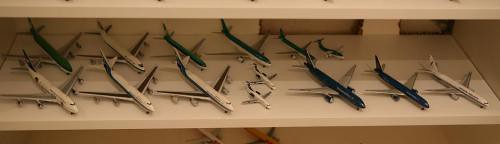The image is a slim, rectangular landscape photo of a white shelf, likely part of a white cabinet or dresser, featuring an array of model airplanes. The shelf displays approximately 14 planes, each angled in the same direction such that their fronts point to the top right and their tails to the top left, providing a side view. These models vary in size, with the majority being around a ruler to half a ruler in length. Three of the planes are smaller, positioned centrally among the larger ones, and they appear to be about half or one third the size of the bigger models. The planes predominantly feature white bodies with blue and red accents, while some models have black or navy bodies with gray wings. The shelf is part of a larger unit, as the contents of another shelf below and parts of yet another above are partially visible. Small bits of additional planes can be seen on the shelf below, indicating a collection that spans multiple shelves.